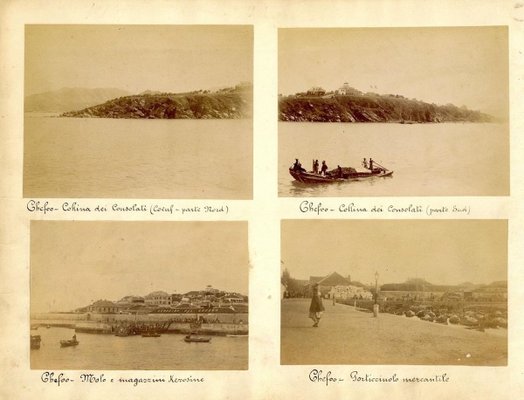This sepia-toned, aged photograph is printed on a card, likely a postcard, and appears to be made on actual photographic paper. The photograph has a detailed grid of four inset images, each bordered in white, with small calligraphic text underneath that suggests it might be in French, potentially describing scenes from a location in Africa. The card shows considerable wear and yellowing, adding to its vintage charm.

The top left image captures a serene water scene with the distant background of an island or rock outcrop. Meanwhile, the top right image features a long, flat boat populated by people against a backdrop of water, suggesting some activity or travel. 

In the bottom left photo, the scene shifts to a bustling shoreline, possibly a very old seaport, lined with multiple buildings indicating a densely built area. Finally, the bottom right photo offers a more terrestrial view with a person walking along what seems to be a walkway near the seaport, distinctively carrying a jar on their head.

Altogether, these four photographs transport the viewer to a distant past with a mix of maritime and coastal life, preserving glimpses of human activity and architectural elements that hint at a unique geographic and cultural setting.